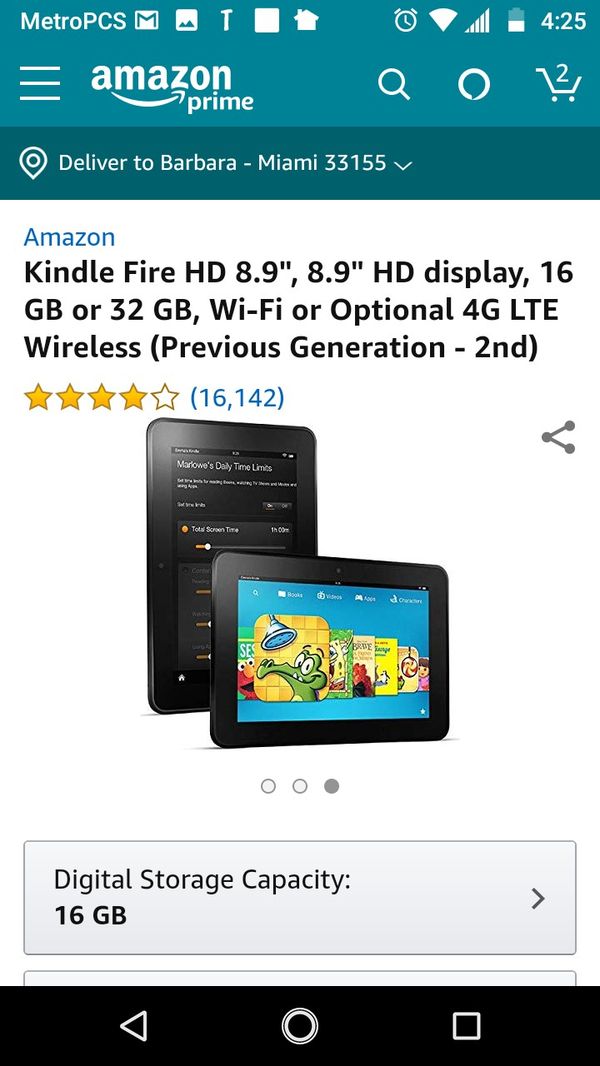The screenshot captures an Amazon product listing viewed on a smartphone, with various icons and details visible from the device's interface. At the top-left corner, there are several icons indicating the phone's carrier, Metro PCS, followed by a Gmail icon, a gallery app icon represented by a white square, and a home icon. On the top-right corner, additional icons display an alarm clock, Wi-Fi signal strength, remaining battery life, and the current time, which reads 4:25.

Beneath these icons, the listing header shows "Amazon Prime" followed by a delivery address: "delivered to Barbara, Miami 33155." The featured product is an "Amazon Kindle Fire HD 8.9 inch," emphasizing the HD display of 8.9 inches. The description mentions availability in two storage options, 16 GB or 32 GB, along with Wi-Fi connectivity and an optional 4G LTE wireless feature. It is further clarified as a "previous generation" device, specifically the second generation.

Finally, the rating section reveals that the product has garnered a four-star rating based on 16,142 customer reviews.